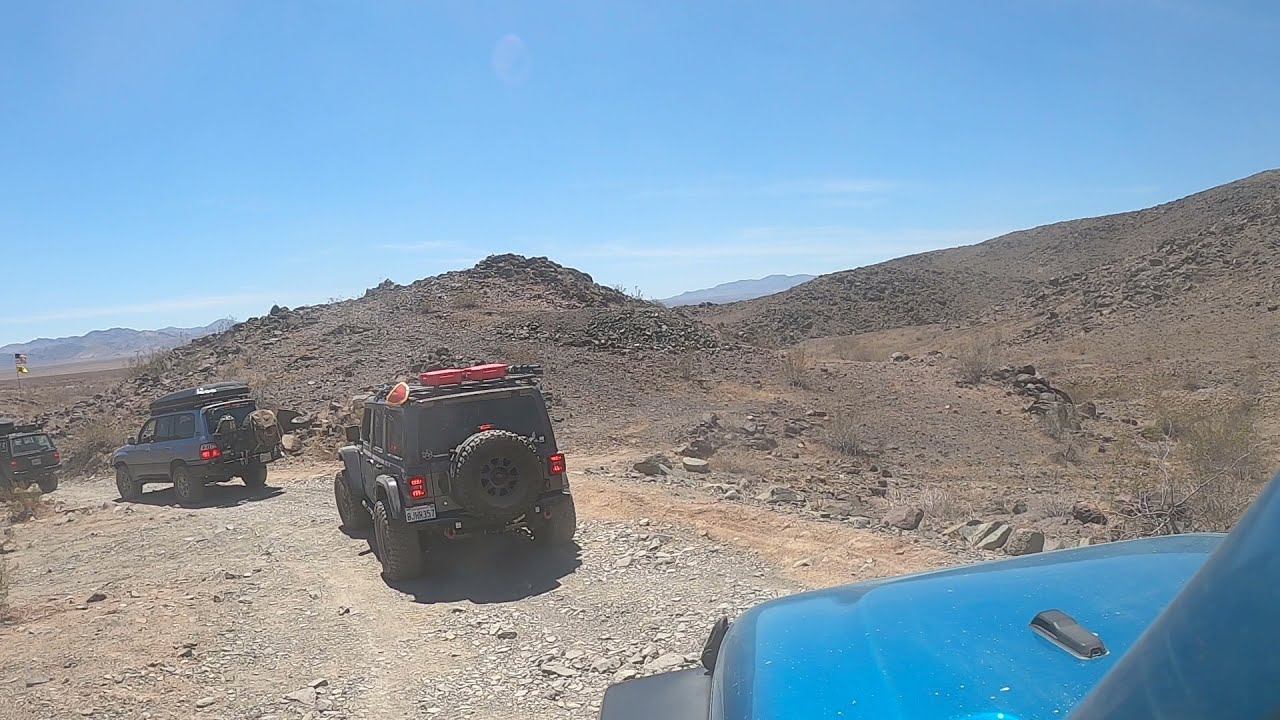In this detailed image, a convoy of off-road vehicles is navigating a rugged mountainous path. The scene is characterized by a dirt and rocky road, with the path composed of mainly brown dirt mixed with white rocks. In the foreground, a blue Jeep is prominently visible, providing the perspective from which the image is taken. The Jeep in front of it is black, equipped with red fuel cans on its roof. Ahead of this black Jeep is a silver SUV with additional cargo on top, followed by another dark-colored vehicle, likely black or dark blue. The vehicles have their rear lights illuminated, suggesting they are moving slowly, perhaps descending the rocky trail. The landscape surrounding the convoy is arid and mountainous, with the closer terrain being sandy and rocky, transitioning to various mountain ranges in the distance. The sky above is a light, clear blue, adorned with various white clouds and a faded moon high atop the image, centered amidst the serene sky. The convoy is on a deserted mountainous trail, reflecting an adventurous outdoor exploration during daylight.